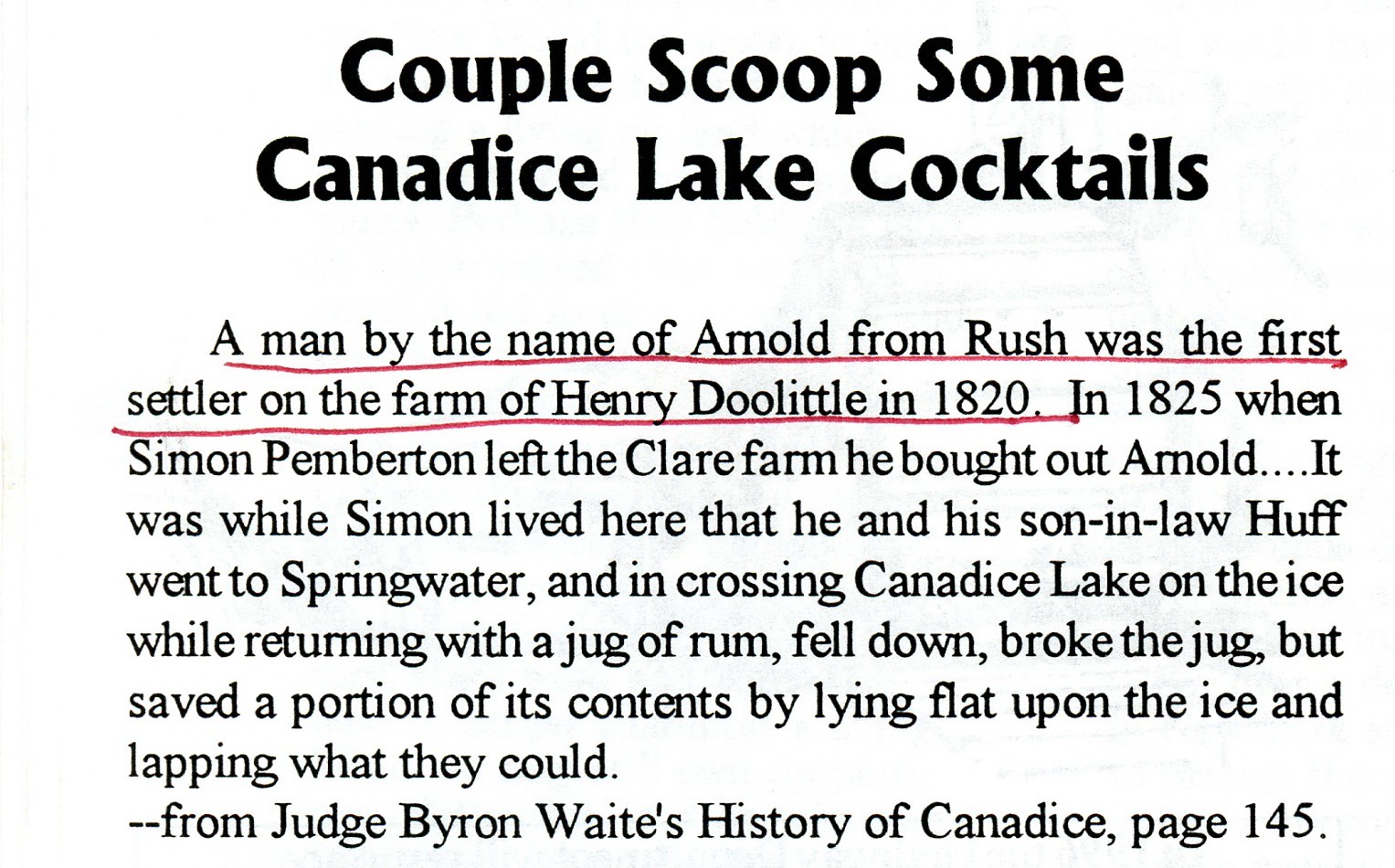The image depicts a block of text against a mostly white background, resembling a newspaper article. Centered at the top in bold, black letters is the title, "Couple Scoop Some Candaice Lake Cocktails." Below the title is a descriptive paragraph in black text. The first sentence, "A man by the name of Arnold from Rush was the first settler on the farm of Henry Doolittle in 1820," is noticeably underlined in red, uneven handwriting. The paragraph continues, detailing how in 1825, Simon Pemberton purchased Arnold's farm and recounting an incident where Simon and his son-in-law Huff fell on the ice of Candaice Lake, breaking a jug of rum but managing to save some of its contents by lying flat and lapping it up. The text concludes with a citation from "Judge Byron Waite's History of Candaice, page 145."